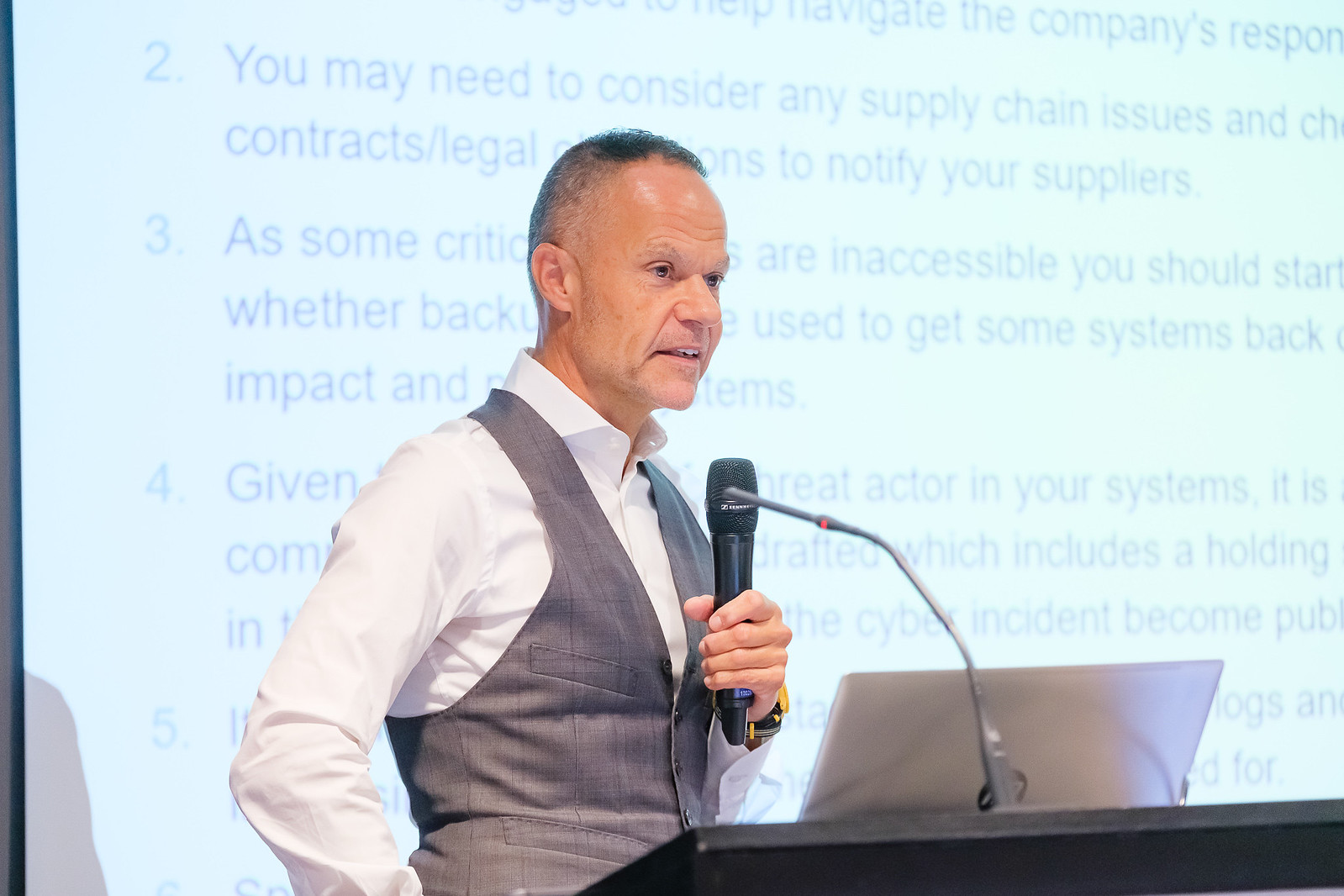The image depicts an older gentleman, likely in his 60s or 70s, standing behind a black podium. He has a lighter skin complexion and short black hair that shows signs of graying. The man is well-dressed in a white long sleeve button-down shirt, slightly unbuttoned at the top, paired with a gray vest. In his left hand, he holds a black microphone, suggesting he is giving a presentation. 

A silver laptop is positioned on the podium in front of him, likely aiding him with his presentation. The background features a clear and well-lit setting with a backboard displaying text, possibly part of a PowerPoint presentation. The legible part of the text includes a list item number two that mentions considering supply chain issues, indicating the topic of his speech. There are no other people visible in the image, and the picture is in color with high clarity.